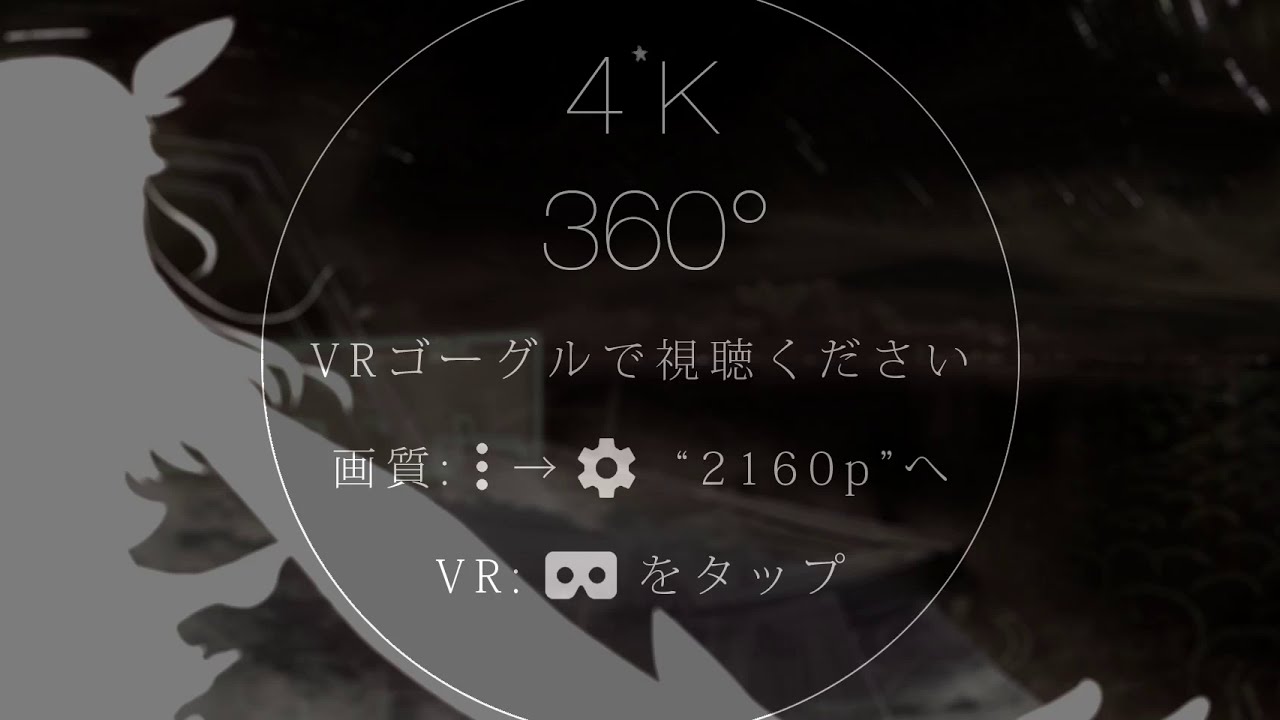This image is a black-and-white, landscape-oriented graphic design, potentially serving as an introduction to a video. The dark background features a grey swirl in the bottom left corner, giving it a slightly abstract, otherworldly feel. Central to the design is a thin white circle encompassing the majority of the image, containing several pieces of technical information. At the top of the circle, the text reads "4K," followed by "360 degrees." Below this are three lines of grey text in a foreign language, possibly Chinese or Japanese, interspersed with various icons including a hamburger menu, three vertical dots, a right-facing arrow, and a settings symbol. Enclosed within apostrophes, the notation "2160P" suggests a video resolution setting. To the left of the circle is an unclear light grey shape, which, along with the geometric patterns behind it, might represent an abstract figure or an anime character outlined in white. The entire composition suggests a high-tech, VR-related video graphic.